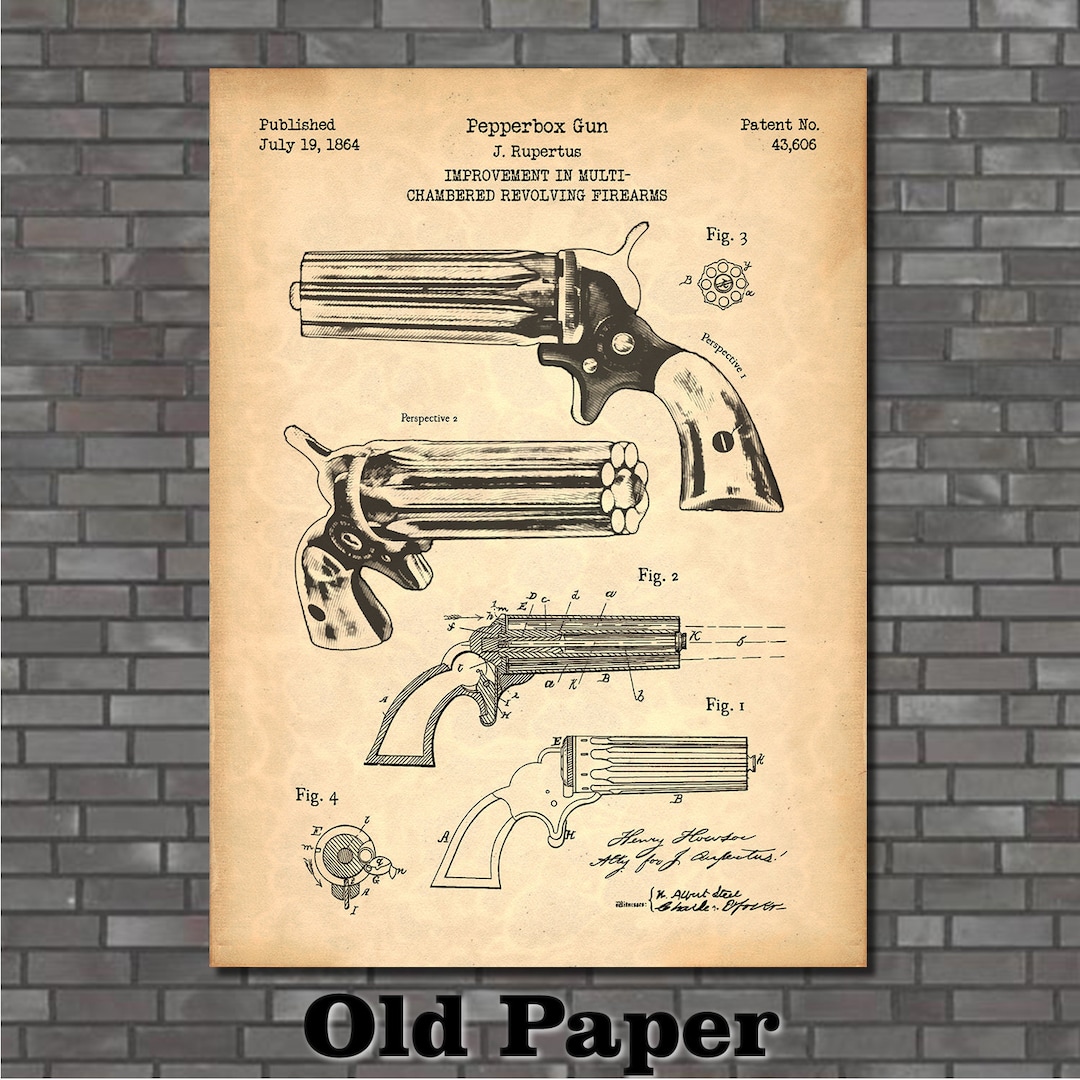This image features a detailed mock-up page of a patent drawing, which appears weathered and aged to simulate old parchment. It is displayed against a slate gray brick wall with a label at the bottom that reads "old paper." The patent, dated July 19, 1864, and numbered 43,606, is for an Improvement in Multi-Chamber Revolving Firearms by J. Rupertis, specifically a Pepperbox gun. The page showcases four meticulous diagrams (Figures 1 through 4) illustrating various angles and internal components of the firearm. These include a side view, a cutaway, and a down-the-barrel perspective, detailing the unique mechanism where six barrels revolve around, rather than a traditional revolving chamber for bullets. Despite the aged appearance of the paper, it is evident this is a carefully crafted reproduction.